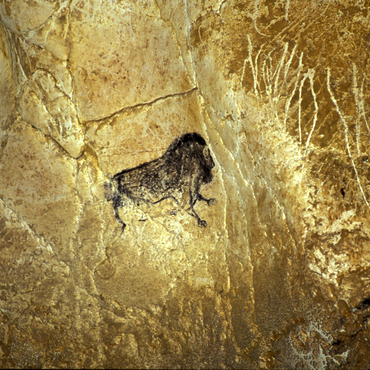The photograph showcases a renowned cave painting discovered in France, set against a vibrant gold to bronze-colored rock wall, which is weathered and ancient. The wall features numerous natural lines, cracks, and etchings, contributing to its timeworn appearance. At the center of the image, there is a small, black figure that experts identify as a musk ox or avobose. The depiction is somewhat ambiguous in form, resembling different animals such as a gorilla, cow, buffalo, pig, or wild boar. The animal appears to be on all fours, with a large, weighty torso and visible front legs, while the back legs seem either unfinished or eroded. The style and context of the drawing evoke connections to ancient civilizations like the Mayans, enhancing its historical and cultural intrigue.